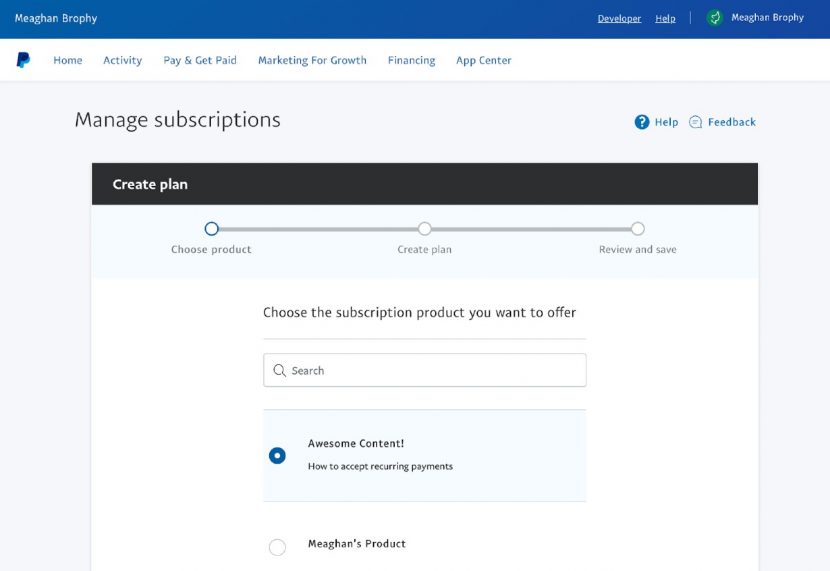The image is a detailed screenshot of a computer screen, showcasing a developer interface. At the top of the screen, a blue banner is prominently displayed, featuring the name "Megan Brophy" on the left, followed by several clickable options: "Developer," "Help," and a green back arrow symbol, which could potentially be part of Megan Brophy's logo.

Below the blue banner lies a white banner with what appears to be a PayPal symbol on the far left. Adjacent to this symbol, a series of menu options are written in gray lettering: "Home," "Activity," "Pay & Get Paid," "Marketing for Growth," "Financing," and "App Center."

Further down, a slightly gray box contains more functionalities, including "Manage Subscriptions," a "Help" button, and a "Feedback" option. Within this gray box, a black banner with white lettering prominently states "Create Plan," flanked by a sliding bar indicating the current step in the creation process: "Choose Product," "Create Plan," and "Review and Save."

Below this, instructions read: "Choose a subscription product you want to offer," accompanied by a search bar for selecting or finding products. Two product options are listed: "Awesome Content," which is selected, and "Megan's Product."

The detailed layout and clear functionality suggest a well-structured, user-friendly interface designed for managing and creating subscription products.